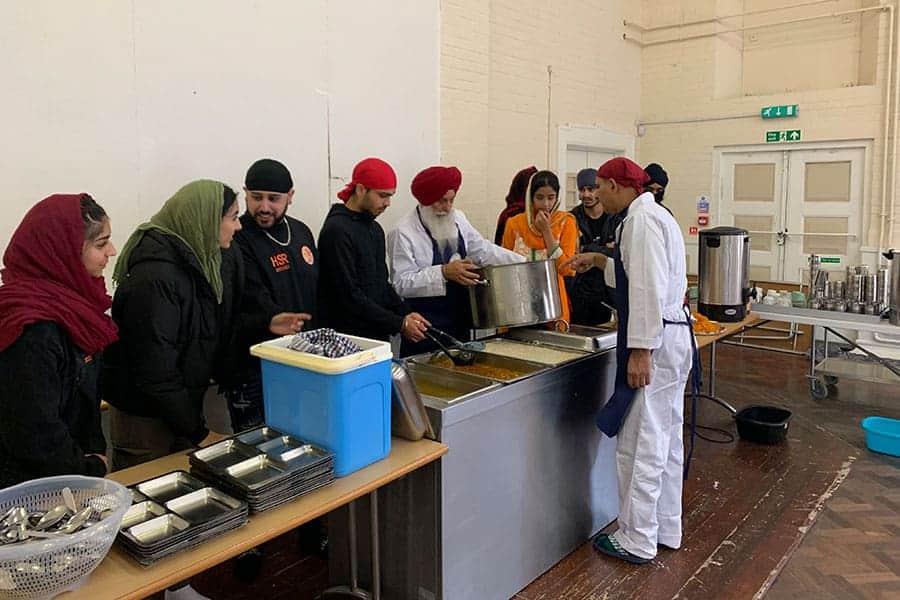The image depicts a busy scene at a soup kitchen, located in a large, utilitarian tan brick building. Men and women, adorned in turbans and brightly colored attire, stand in line, awaiting their turn to be served. A long, brown table holds food trays, a bowl of silverware, and a blue cooler at one end. Further along the line, a gray serving table features several silver serving dishes. Two chefs, one in a blue apron with a burgundy headdress and the other in a white coat with a black apron and red headscarf, are serving food from a large silver pot. The chef in the blue apron points at the pot, seemingly giving instructions. An additional table on the opposite side of the room holds more silver serving dishes on the floor, accompanied by a black pan and a blue pan. The eclectic mix of head coverings, facial hair, and the complexions of the people suggest the scene may take place in the Middle East or India. The room is equipped with all necessary items, including stacks of metal trays and a coffee machine, providing a sense of organized, community-driven service.